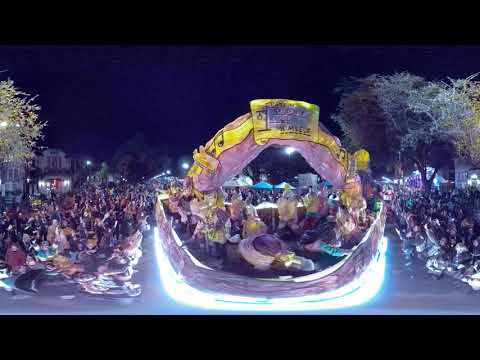The image captures a vibrant night parade, prominently featuring a brightly lit float moving down a road flanked by crowds of people. The horizontal rectangular picture has black strips at the top and bottom, framing the nighttime scene. The sky is pitch black, accentuating the festive atmosphere. On both sides of the road, spectators are seated, with some standing behind them near trees and possibly distant buildings. At the center of the image, the float stands out, adorned with an arching design in soft purple and yellow, and illuminated from below. Although the text on the float is illegible, a yellow banner with black music symbols can be seen above it. Behind the float, there are small umbrellas, whose exact placement is unclear due to the image's blur. The entire scene is bathed in a mix of blue, white, and multicolored lights, highlighting the joyous occasion that might resemble an outdoor festival or possibly even a painted depiction, given the blending of colors and indistinct features.